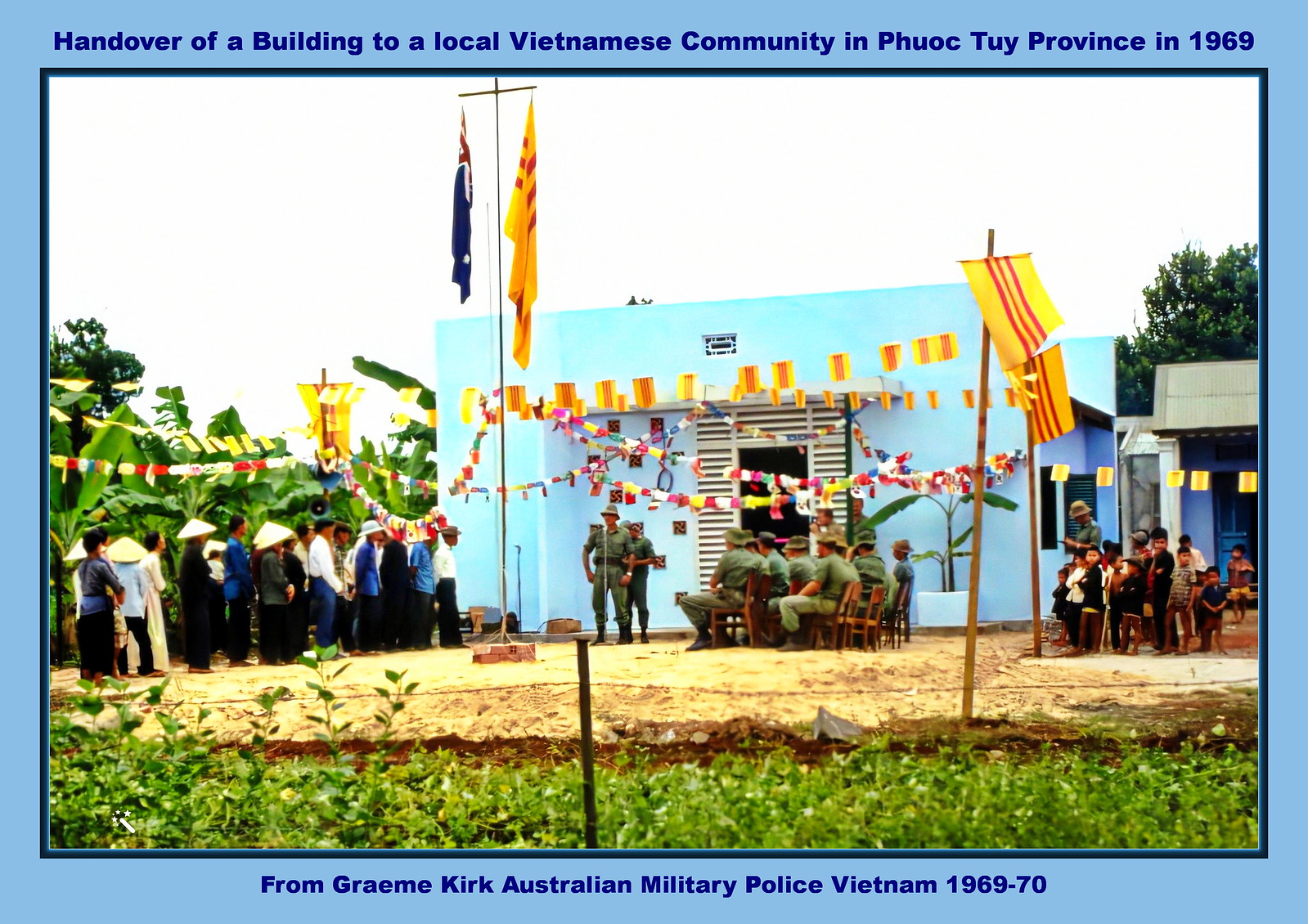This color photograph, bordered in blue, captures an outdoor scene marked by a significant event in 1969. The image bears the heading "Handover of a building to a local Vietnamese community in Phuoc Thuy province in 1969" at the top, and the footer reads "From Graham Kirk, Australian Military Police, Vietnam 1969-70." Central to the photograph is a light blue, almost turquoise, rectangular building adorned with a string of yellow and red flags. Atop the building, several flags are also visible. Below, a dozen men in green military uniforms are seated on brown wooden chairs, with two standing among them, facing the camera.

To the far left, a line of local Vietnamese men and women, dressed in traditional attire including conical hats, stands attentively. Off to the right, a small group of children can be observed, also standing. The foreground of the image shows green vegetation, including leaves, trees, and ferns, adding a contrasting touch of nature against the mainly yellowish dirt area directly in front of the building. This image, almost postcard-like, captures a poignant moment of cultural and community exchange during the Vietnam War.